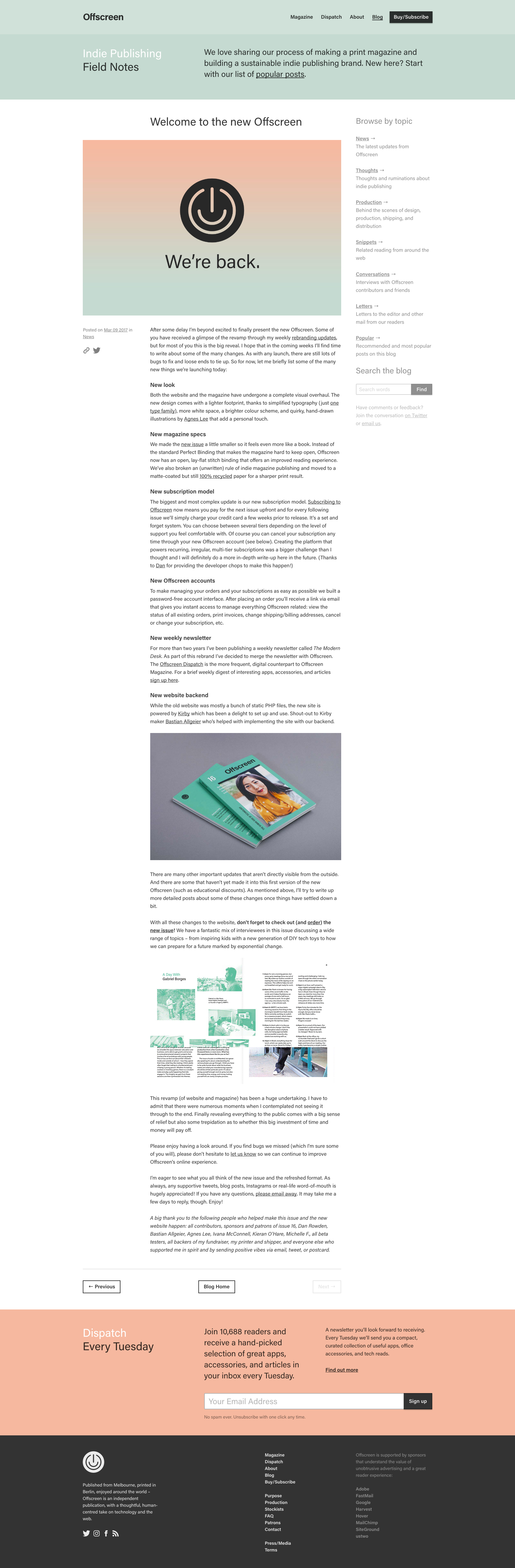**Offscreen's Grand Relaunch**

Welcome to the newly revamped Offscreen! After some delays, we are thrilled to present the much-anticipated makeover. For those who have been following our weekly rebranding updates, you may have caught glimpses of this transformation. For others, this is the grand reveal. Over the coming weeks, I hope to write more in-depth about the significant changes we've implemented. As with any major launch, there are still bugs to fix and loose ends to tie up. But for now, let me introduce you to the exciting new features of Offscreen.

**New Look:** Both the website and magazine have undergone a complete visual overhaul. The new design boasts a lighter footprint with simplified typography, using just one type family, more white space, a brighter color scheme, and quirky hand-drawn illustrations by Agnes Lee that lend a personal touch.

**New Magazine Specs:** The new issue is slightly smaller, enhancing its book-like feel. We’ve shifted from the standard perfect binding to an open, lay-flat stitch binding for an improved reading experience. Breaking the norms of indie magazine publishing, we’ve opted for matte-coated yet 100% recycled paper, resulting in sharper print quality.

**New Subscription Model:** Our most complex update is the new subscription model. Subscribers now pay upfront for the next issue, and for each subsequent issue, your credit card will be charged a few weeks prior to release. It’s a set-and-forget system with several support tiers to choose from. Subscriptions can be canceled at any time through your new Offscreen account. Creating a platform for recurring, irregular, multi-tier subscriptions was a bigger challenge than anticipated—more details to come. Special thanks to Dan for his development expertise in making this happen.

**New Offscreen Accounts:** For easy order and subscription management, we’ve built a password-free account interface. After placing an order, you’ll receive an email link providing instant access to manage all things Offscreen—view order statuses, print invoices, change addresses, and adjust subscriptions.

**New Weekly Newsletter:** We've merged "The Modern Desk" newsletter with Offscreen. Now called "The Offscreen Dispatch," it offers a weekly digest of interesting apps, accessories, and articles. Sign up to stay informed.

**New Website Backend:** Transitioning from static PHP files, our new site is powered by Kirby, which has been a pleasure to set up. Thanks to Kirby maker Bastien Allagier for helping with the implementation.

Beneath this text is an image displaying two Offscreen magazines. The cover features an Asian woman with long black hair and red lipstick, wearing a mustard yellow scarf with white polka dots. Underneath, I mention that there are numerous important updates, some invisible from the outside, and others not yet included in this version, like educational discounts. More detailed posts about these changes will follow as things settle.

Don't forget to check out and order the new issue! It includes a fantastic mix of interviews discussing topics from inspiring kids with new DIY tech toys to preparing for a future marked by exponential change.

This revamp of our website and magazine has been a huge undertaking. There were moments of doubt, but finally revealing it to the public is both a relief and a source of apprehension about whether the investment will pay off. Please explore, and if you find any bugs, let us know so we can improve Offscreen’s online experience. Your thoughts on the new issue and format are eagerly awaited. Supportive tweets, blog posts, Instagrams, or word of mouth are hugely appreciated.

A huge thank you to everyone who made this possible: contributors, sponsors, patrons of Issue 16, Dan Roden, Bastien Allagier, Agnes Lee, Ivana McConnell, Kieran O'Hare, Michelle F., all beta testers, fundraiser backers, our printer and shipper, and everyone else sending positive vibes. Enjoy the new Offscreen!

**Dispatch:** Every Tuesday.